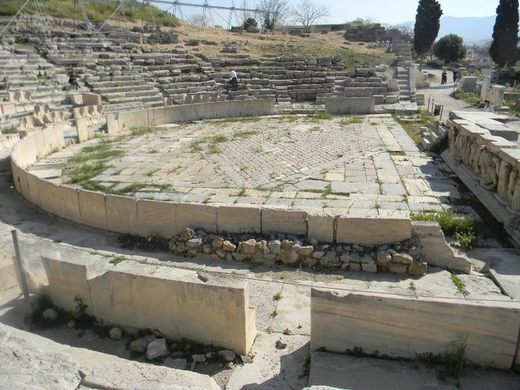This photograph captures the ruins of an outdoor Roman amphitheater, possibly ancient but clearly in a state of disrepair. The amphitheater is semi-circular in shape, characterized by degraded stone seating that curves in a horseshoe-like formation around what likely used to be the stage area. The stones, primarily gray-tan in color with a limestone or sandstone texture, are broken and crumbled, some piled haphazardly around the site. The central stage area features inlaid brick, adding to the historical ambiance of the scene. Tall trees and distant mountains provide a scenic backdrop, with one person seen walking through the ruins, adding a sense of scale to the photograph. The image, taken in daylight, exudes a timeless quality, capturing the enduring legacy of what might have been a grand arena or a coliseum, perhaps indicative of historical sites found in regions like Italy or Greece.